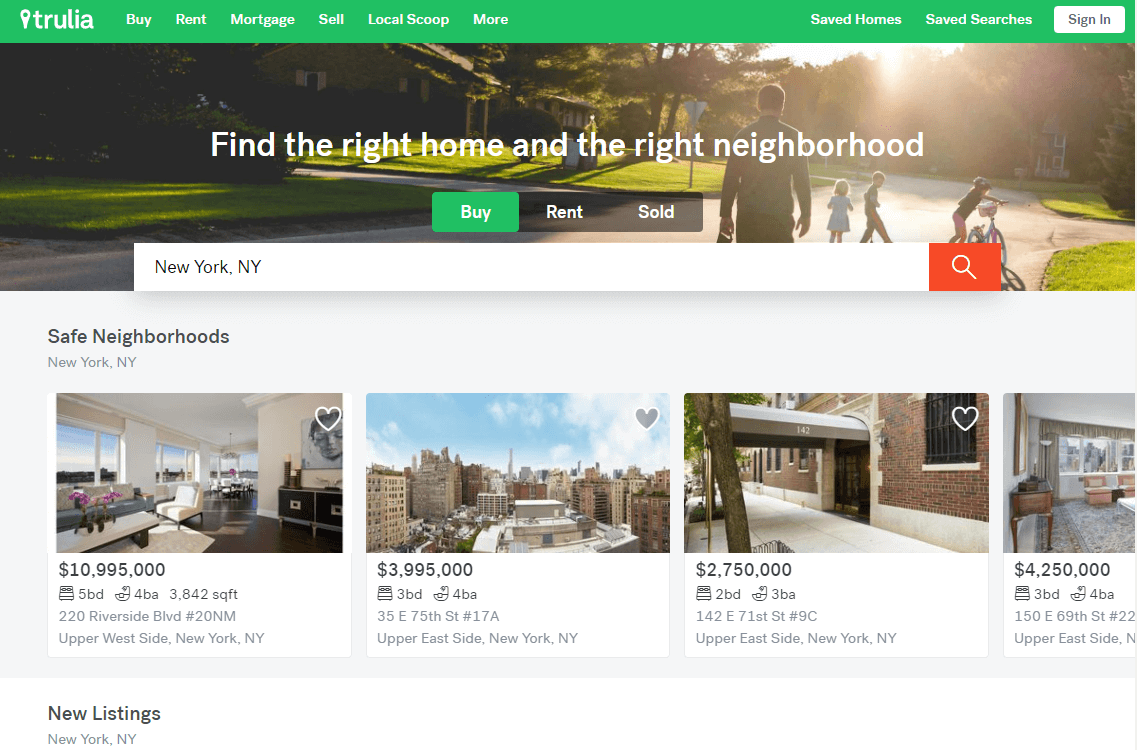Screenshot of the Trulia Website Interface

At the top of the screenshot, the Trulia logo is prominently displayed in the upper left corner. The navigation bar, which spans from left to right and is highlighted in green, features white text with the following options: Buy, Rent, Mortgage, Sell, Local Scoop, More. On the right side of this green bar, there are additional options including Saved Homes, Saved Searches, and a Sign In button located in the very top right corner.

Below the navigation bar, a visually engaging banner features an image of a man strolling down a neighborhood street with several children, presumably his own. This picturesque neighborhood is adorned with large evergreen trees in the front yards of prominent, luxurious homes. Superimposed over this image, in bold white letters, is the tagline: "Find the Right Home in the Right Neighborhood."

Directly beneath the tagline, there are three interactive buttons: a green “Buy” button, alongside gray “Rent” and “Sell” buttons, indicating the focus is currently set on buying properties. Below these buttons sits a search bar pre-filled with "New York, New York City, New York," accompanied by an orange search button to the right of the bar.

Further down, a section dedicated to "Safe Neighborhoods" in New York, New York is introduced. This section features four property listings with corresponding images and monthly rental prices displayed below each image. The listings are as follows: $11,000/month, $4,000/month, $2,750/month, and $4,250/month, shown from left to right.